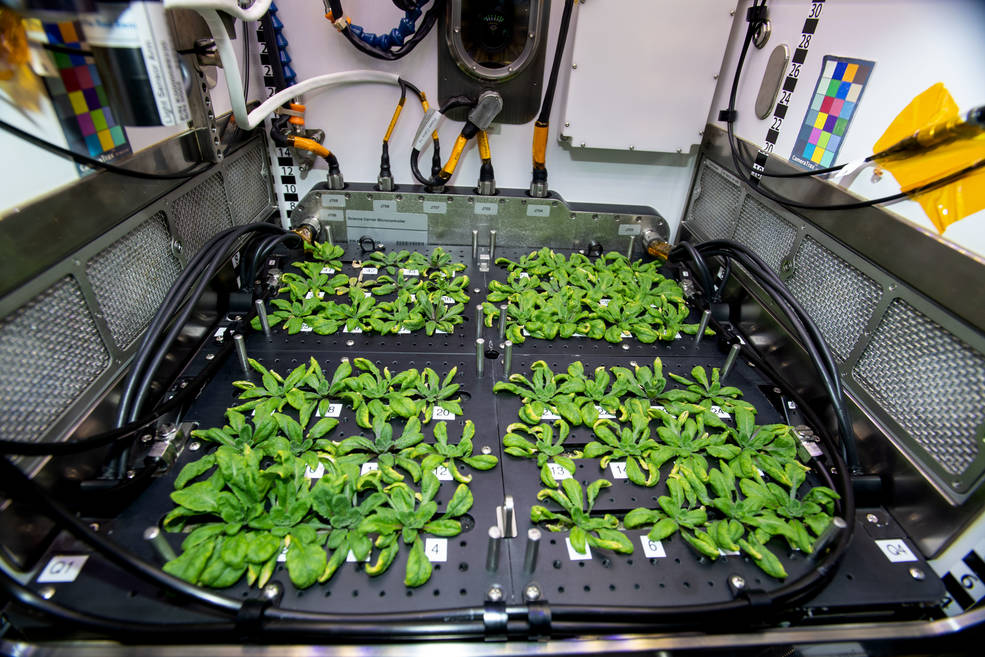The image depicts a sophisticated plant cultivation system featuring a black plastic tray divided into four sections. Each section contains small patches of green plants with light curling leaves, some of which exhibit yellowing, indicative of the natural aging process. The tray has multiple cutout circles and appears flat and opaque, resembling a strainer. Numerous black cables and hoses, which emanate from the tray and connect to a mechanical device with a silver connector, surround the plants and run in all directions. This mechanical device seems to interface with the surrounding environment via cords connected to the wall. Additionally, there are rectangular panels on both the left and right walls, each displaying rows of colored squares and numerical sequences, some partially obscured by cords. The technology-intensive setup suggests a methodical approach to plant growth, possibly involving advanced control systems.